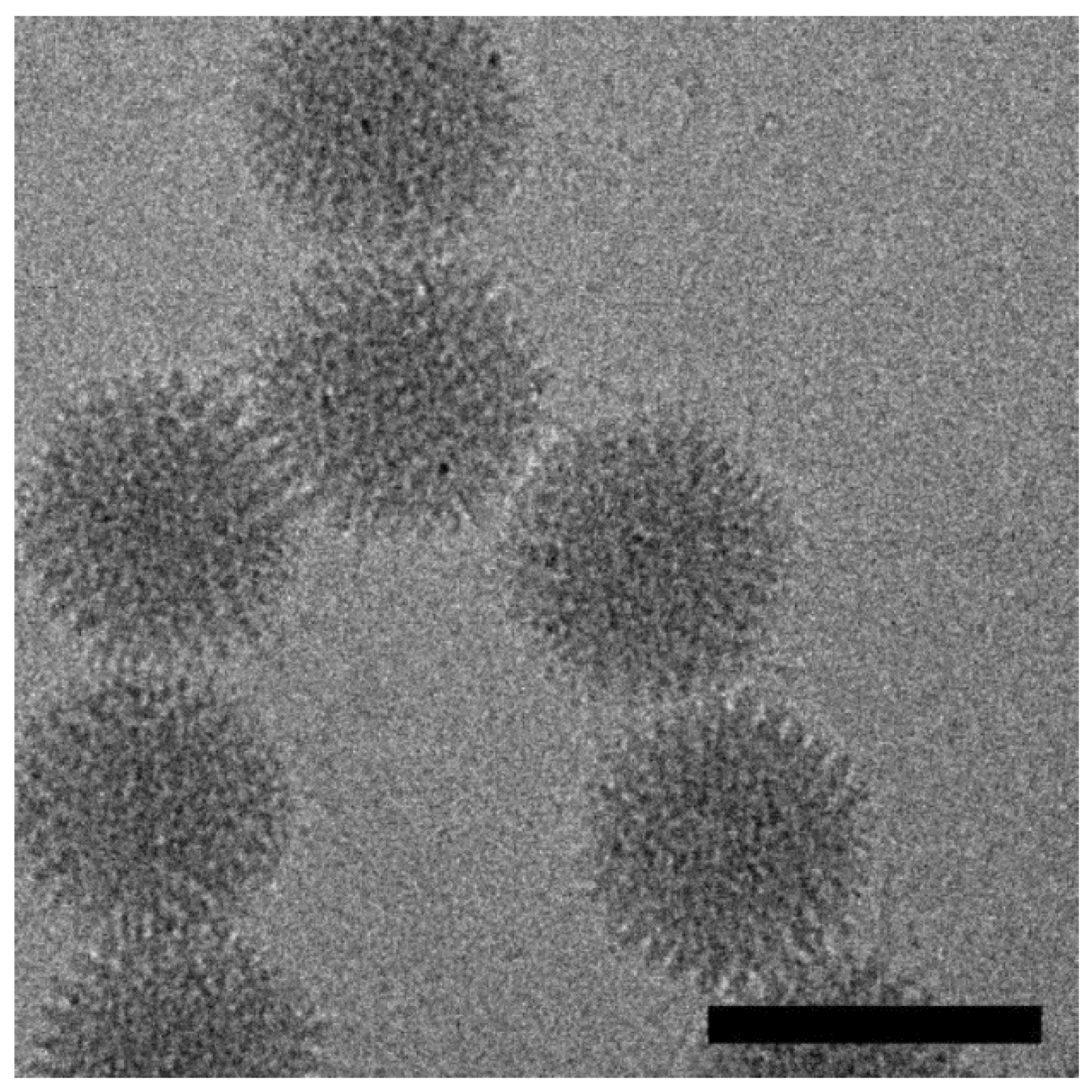The image features a medium gray, textured background that gives the appearance of fabric or a scientific slide. Scattered across this grainy, sandy-looking backdrop are several circular and spiky shapes, resembling cells or germs. These shapes are in varying shades of gray with darker specks at their centers and lighter specks around their edges, reminiscent of microscopic views or images of the coronavirus. There are approximately seven to eight of these clusters that stand out against the gray background. Additionally, at the bottom right corner, a long, narrow black rectangular box appears, which seems to obscure or highlight a portion of the image. The overall scene is highly detailed, giving a tactile impression, as if the textured background and the spiky shapes could be felt if touched.